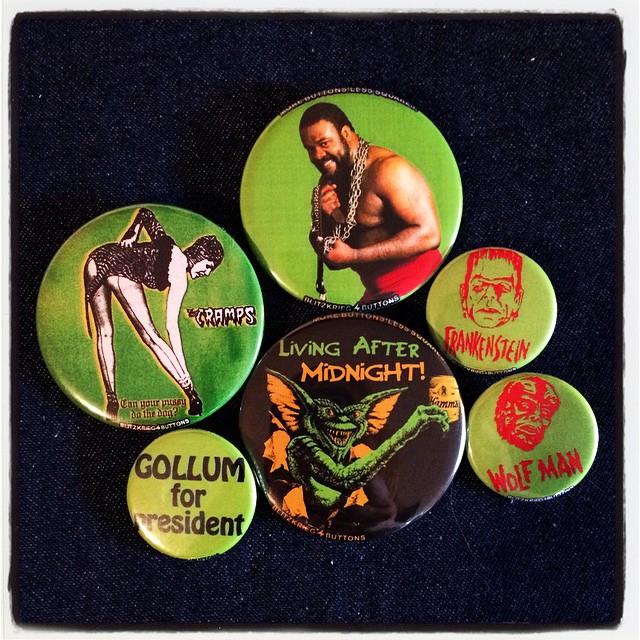In this photograph, we see six circular pin-back buttons of varying sizes arranged on a dark blue, denim-like surface with tiny white dots. Three of these buttons are larger, while the remaining three are smaller. Starting with the larger buttons, one features a photograph of a dark-skinned, shirtless man wearing a heavy chain around his neck and red trunks. Another larger button, marked with the word "C-R-A-M-P-S," displays an image of a woman in a black and white leotard, bending over with a pose that suggests she might have animalistic features, including what appears to be a tail. Next, we find a nostalgic design of a gremlin from the movie "Gremlins" on a black button, with text saying "Living After Midnight." 

As for the smaller buttons, one is light yellow and promotes "Gollum for President," referencing the character from "The Lord of the Rings." Another smaller button depicts Frankenstein's monster with the word "Frankenstein" in red against a yellow background. The final button features an illustration of a wolfman, with the word "Wolfman" in red against a light green background. Collectively, these buttons reflect a mix of pop culture themes and vintage aesthetics, all neatly arranged on a textured background.